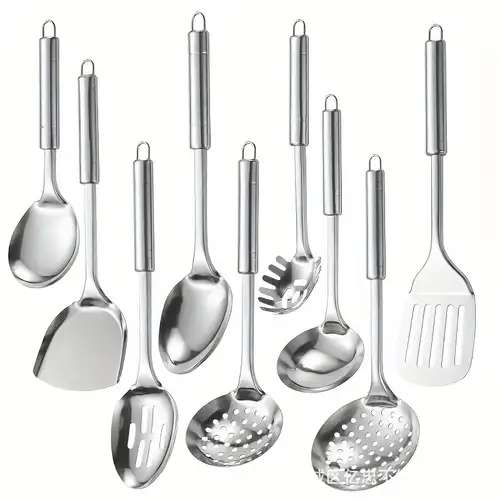This artist’s black and white sketch intricately illustrates nine vertically arranged stainless steel cooking utensils, each suspended as if hanging from a rack. On the far left, there's a large ladle with a wide, circular bowl. Next is a flat, scooping spatula. Positioned to its right is a slotted spoon with elongated vertical holes. Following is a regular large spoon with an oval-shaped bowl. Above and to the right is a colander spoon with perforations for draining. Adjacent is a spaghetti-serving spoon, identifiable by its wide tines for picking up pasta. Positioned next to it is another ladle, larger with a deeper bowl. Further right is a second colander spoon with a wider perforated circle, designed for straining. Finally, on the far right, there’s a thin spatula with multiple vertical slots. The detailed rendering, likely using pencil or charcoal, emphasizes the realistic and metallic texture of these kitchen tools, showcasing their varied and specific uses.